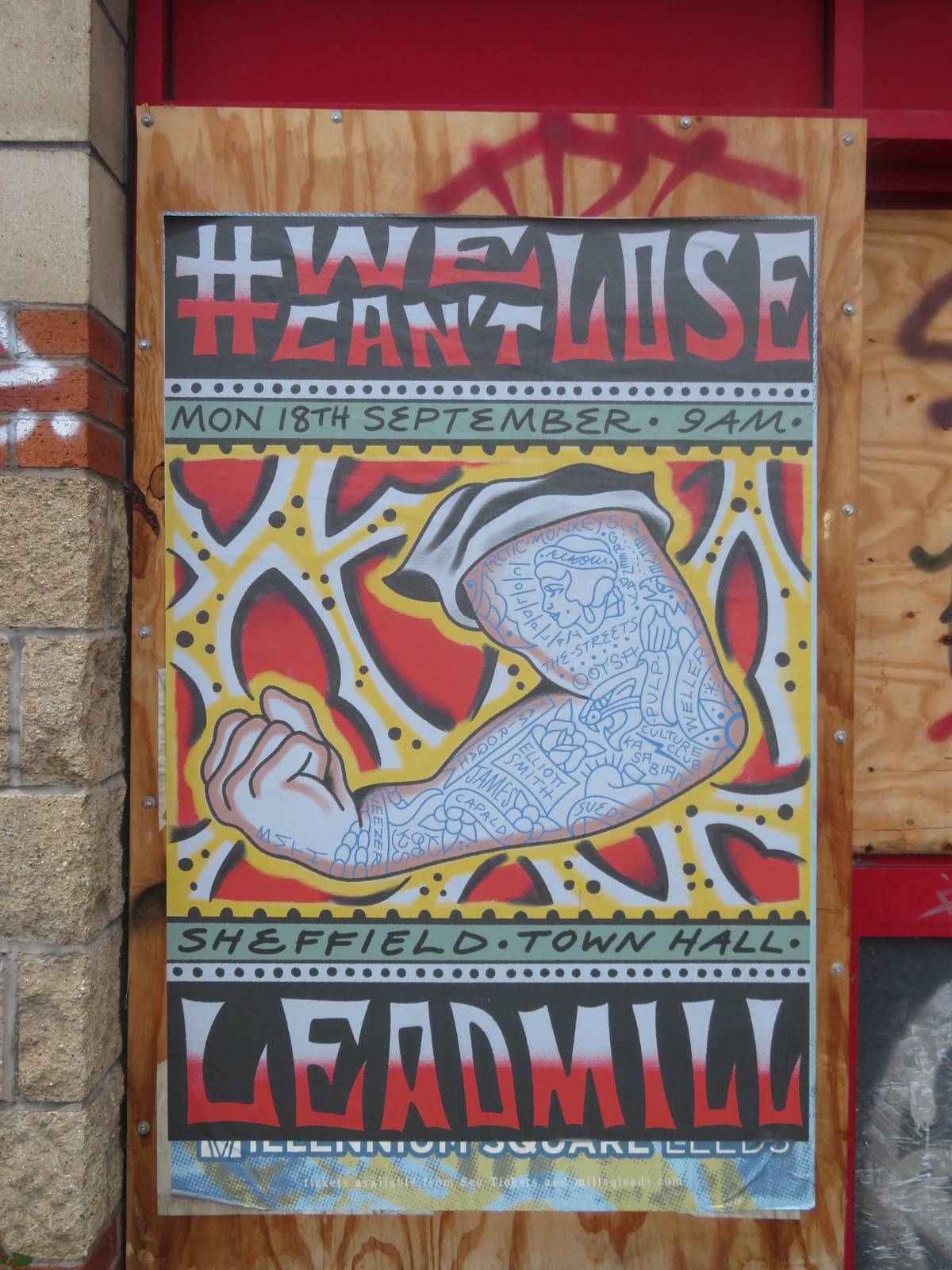The image depicts an artistic, hand-drawn poster mounted on a plywood panel covered in graffiti, with a backdrop of red wood and exposed brick. The poster, reminiscent of a tattoo artist's work, is vibrant with red, white, black, and yellow hues. Dominating the design is a flexed arm adorned with a tattoo sleeve that includes names, a woman's head, and streets, set against a red, white, and yellow background.

At the top of the poster, bold red and white letters spell out "#WeCan'tLose" against a black striped background with white dots. Just beneath, a green stripe announces "Monday, 18th September, 9 a.m." followed by the striking image of the tattooed arm. Further down, another green stripe reads "Sheffield Town Hall," leading to more dotted white space and ending in a black strip that states "Leadmill" in white and red lettering.